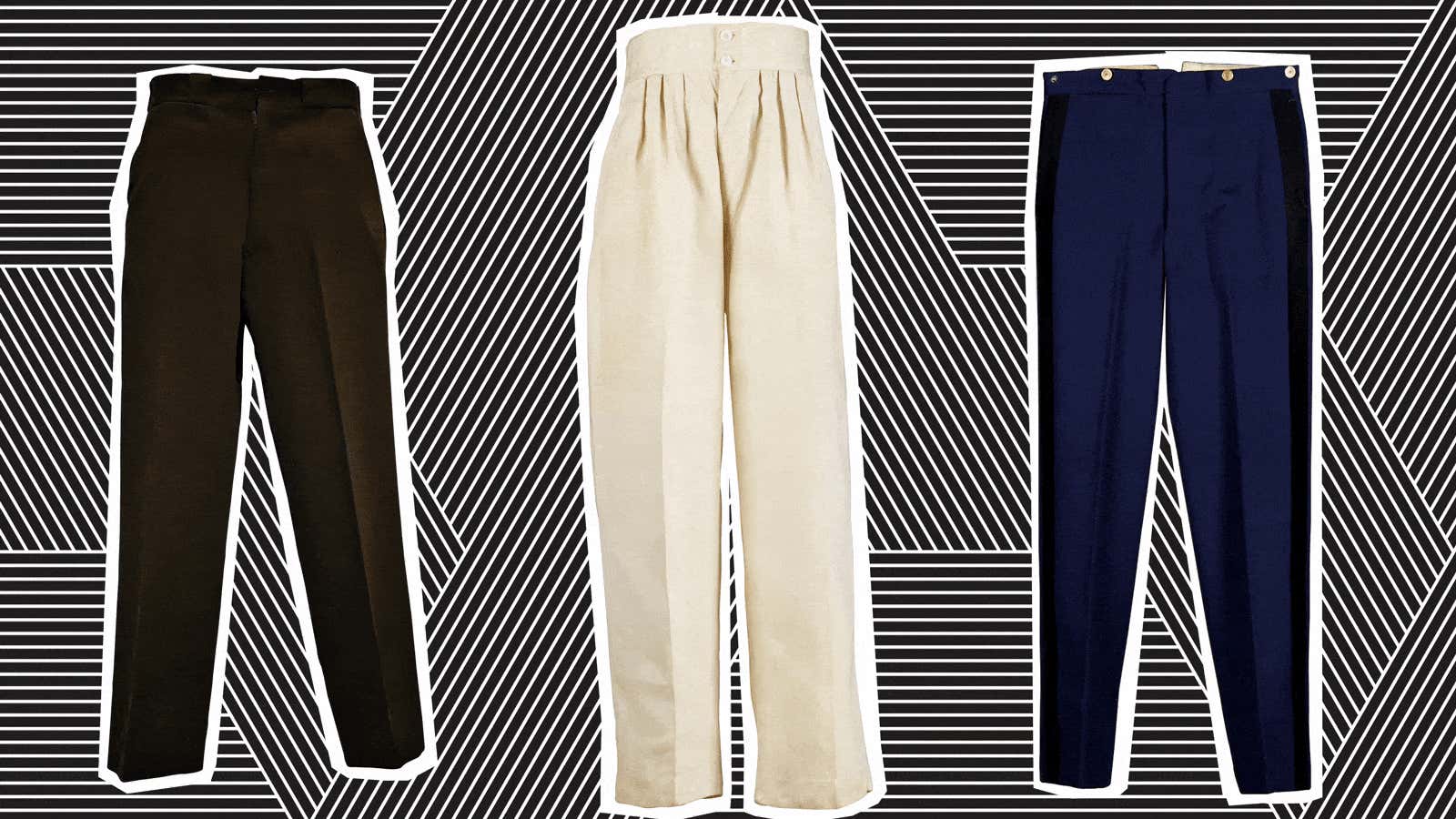In this striking image, three pairs of pants are displayed against a dynamic black and white striped background, where thin lines run in various directions. The pants, each outlined in white to make them stand out, are evenly spaced across the composition. On the left, there's a pair of black pants featuring an ironed line running down the middle of each thigh. The center showcases high-waisted, light gray or cream-colored pants with pleats and two buttons at the top, giving them a ruffled appearance. On the right, the dark blue, slim-fitted pants also feature an ironed line and two gold buttons on each side, adding a touch of elegance. The contrasting colors and the intricate background design create a visually appealing and organized presentation.